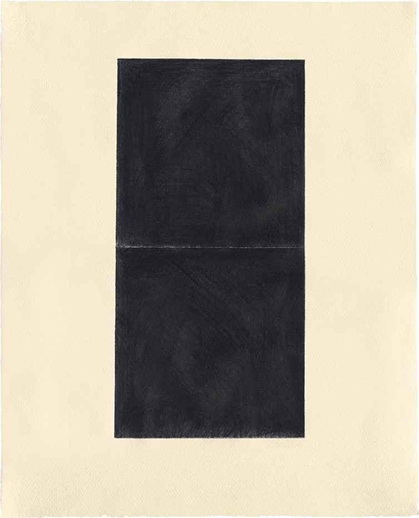The image depicts a modern art piece set against a light, flesh-toned background, resembling a faded cream or pinkish beige canvas. The centerpiece of this artwork is a large, black rectangle that dominates the upper half of the composition. This black rectangle isn't uniformly painted; it features subtle gray swirls and splotches throughout, giving it a weathered, brushed appearance. A prominent white line cuts vertically down the center of the black rectangle, suggesting it has been folded in half and then flattened out again. The contrast between the dynamic, textured black rectangle and the muted, monochromatic background creates a striking visual. The background appears brighter and more distinct around the edges, further emphasizing the black rectangle's central position and adding depth to the piece.